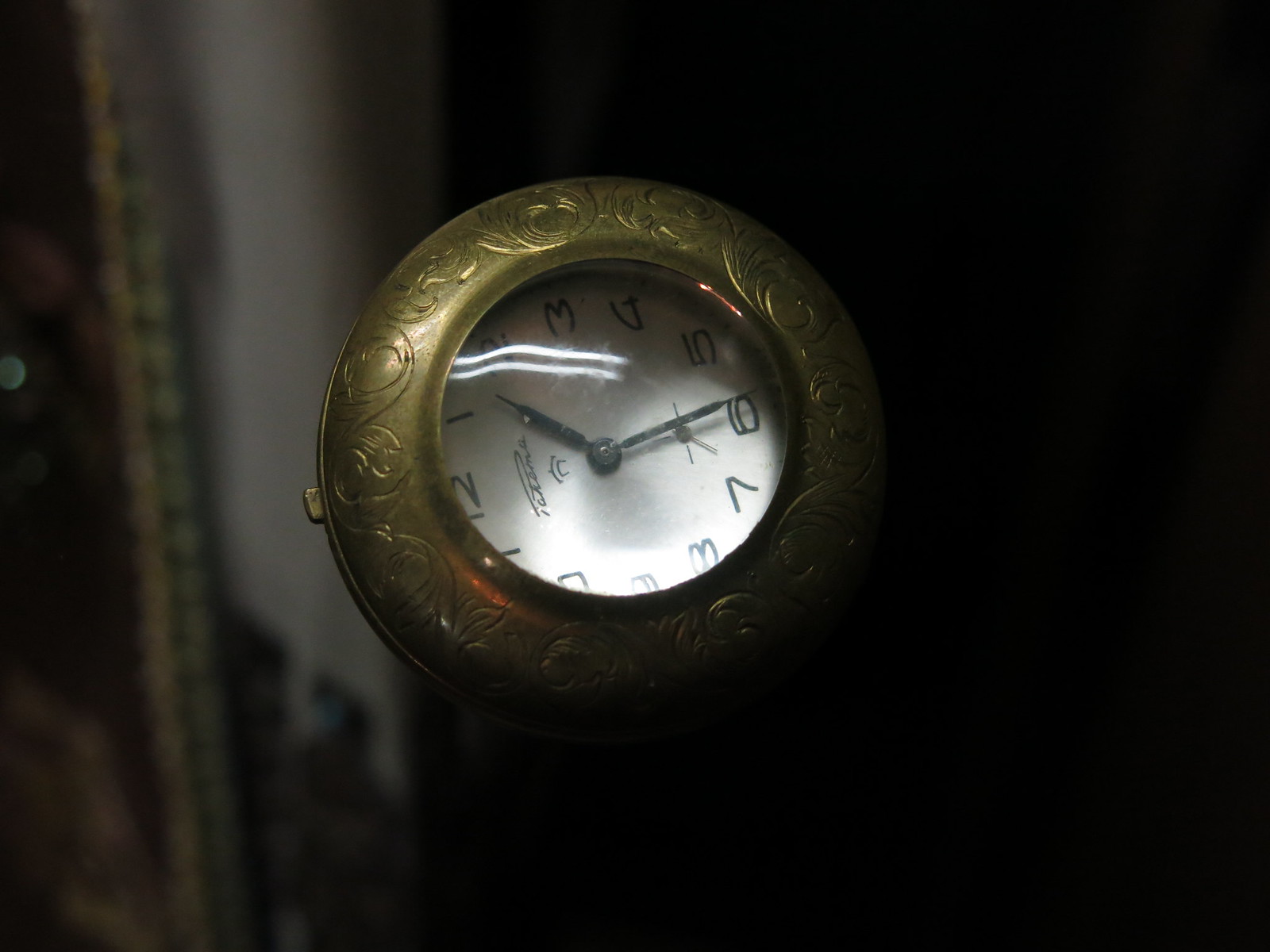This is a photograph featuring a roundish, brass or gold-colored alarm clock centrally positioned within a dark setting. The clock, resembling a pocket watch, has a gold casing adorned with a leaf or vine design on the upper portion. The white clock face displays 12 black Arabic numerals, from 12 to 11, with an unreadable inscription. The black minute and hour hands indicate the time as 1:29. The clock is positioned against a backdrop that combines dark and light elements: a predominantly black area suggesting a dark room or shelf, transitioning into a grayish section. Behind the clock is a whitish wall with the lower edge of a golden picture frame visible, likely surrounding a painting or photograph. The frame contains touches of green and possibly brown or pink hues, though the exact content of the image within the frame remains indiscernible. A small golden dial on the left of the clock's top is visible, presumably for adjusting the time.